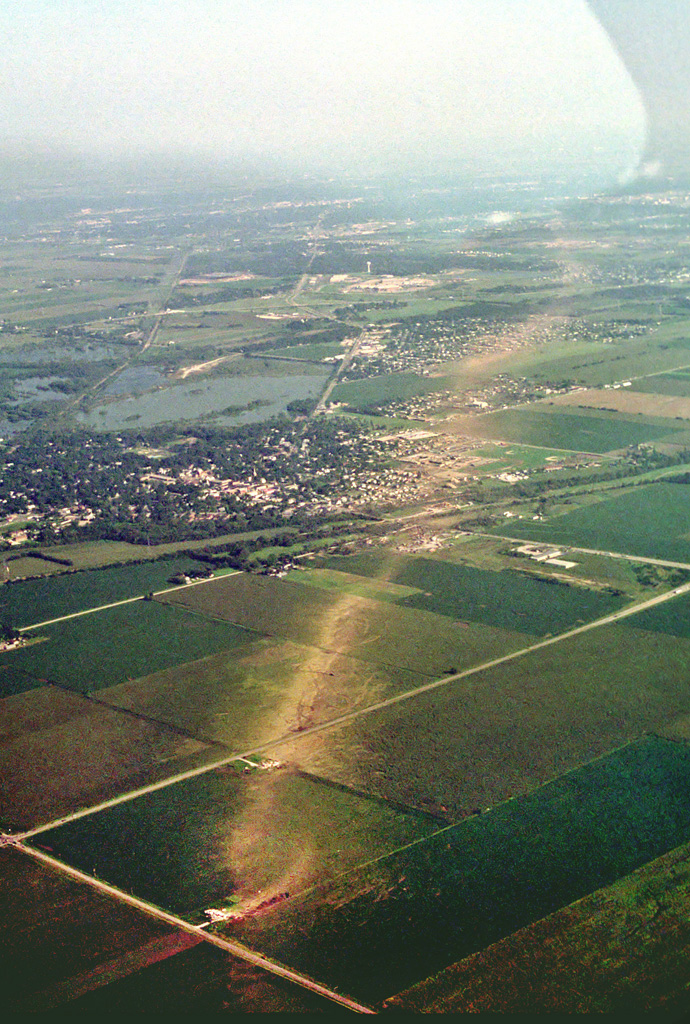This detailed aerial photograph, seemingly taken from an airplane window, captures a varied landscape with vivid detail. The lower portion of the image showcases large, rectangular farm fields in different shades of green, bordered by intersecting dirt roads that create a patchwork effect across the ground. Scattered among these fields are lighter brown and reddish areas, indicating perhaps different types of crops or barren patches.

Beyond these agricultural sections lies a small town or village, characterized by scattered small buildings and houses nestled among dense clusters of dark green trees, which provide a stark contrast to the orderly fields. Farther in the distance, a water body, likely a pond or small lake, filled with blue water, can be seen reflecting the sunlight. The horizon reveals an additional expanse of land, transitioning smoothly into the sky, which is dotted with clouds and lit by the sun, adding a natural shading effect to different parts of the terrain. A subtle glare across the image suggests the sun's reflection off the airplane window, enhancing the photograph's authenticity and providing a sense of height and perspective.